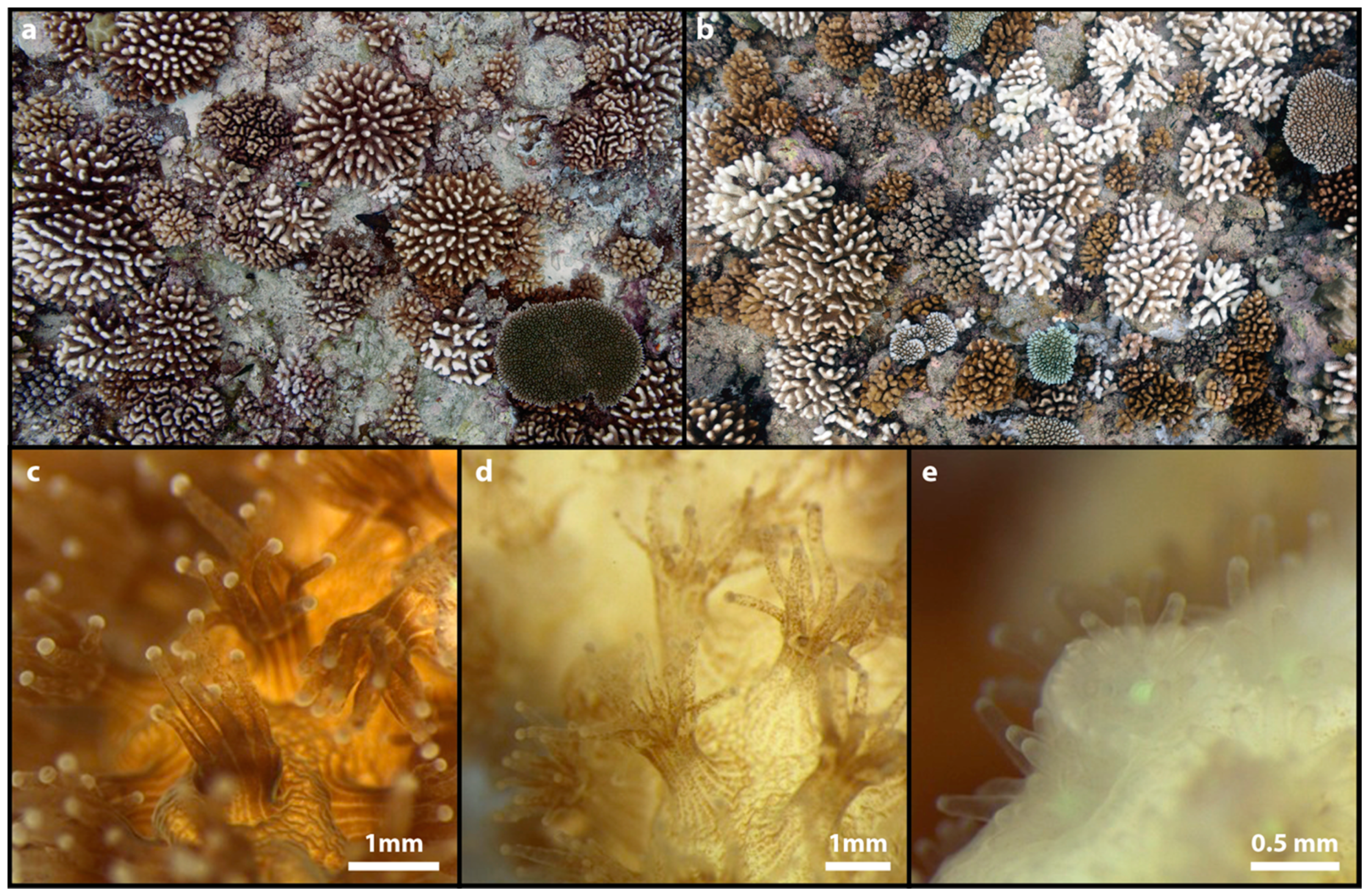The image is divided into five sections, with the top half split into two parts labeled A and B, and the bottom half into three parts labeled C, D, and E. The scene depicts various underwater growths resembling those found on coral reefs or rocks, viewed from above. Sections A and B showcase snow-covered, dark brown, yellow, and white puffy ball-like sea plants, possibly pine cones and mushrooms or fungus, mixed with some green leaves in A and another leaf in B. Section C features a blurred, golden and white image with little white specks of flowers and other golden blooms, marked 1mm at the bottom and labeled C at the top. Section D, also marked 1mm at the bottom, shows a tan and gold swirly and blurred image labeled D. Finally, Section E illustrates white, tentacle-like structures labeled E at the top, with 0.5mm at the bottom. The overall palette transitions from dark brown to light brown, white, creamy, and some greenish hues, resembling coral reef anemones with finger-like, spongy growths.